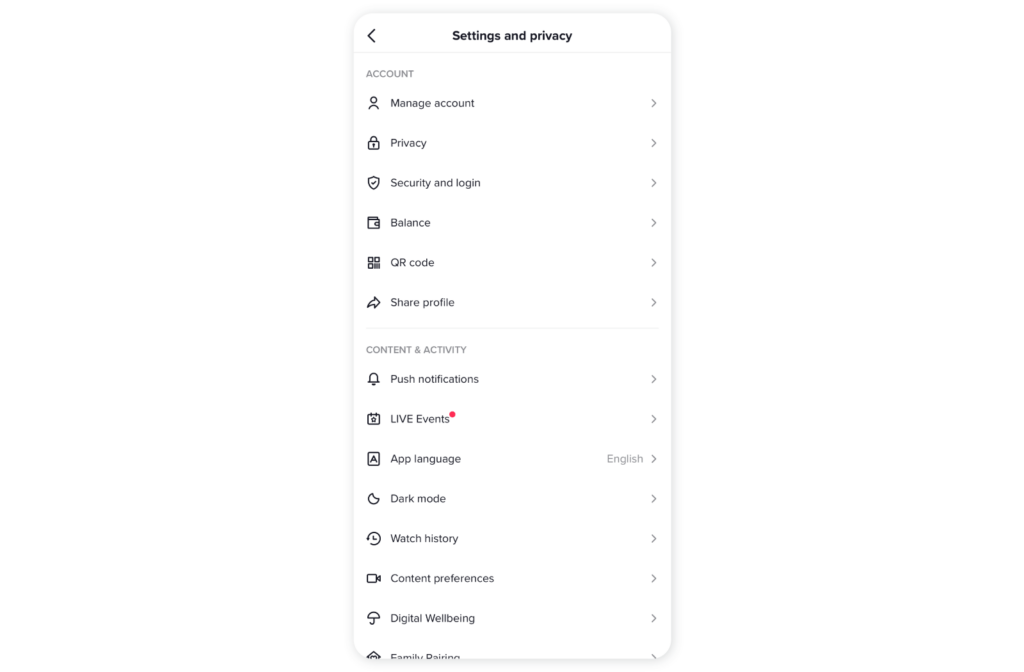This image is a clean, high-quality screen capture with a white background and black font, featuring various black icons and descriptive text. At the top, there's a black arrow followed by the text "Settings and Privacy." Below, the section titled "Account" is in gray, serving as a heading for a list of options, each accompanied by corresponding icons and gray arrows. 

1. **Manage Account**: Represented by a person icon.
2. **Privacy**: Indicated by a padlock icon.
3. **Security and Login**: Shown with a shield icon featuring a check mark.
4. **Balance**: Illustrated by a wallet icon.
5. **QR Code**: Depicted with a pattern of black squares.
6. **Share Profile**: Accompanied by an arrow icon.
7. **Push Notifications**: Marked with a bell icon.
8. **Live Events**: Characterized by a calendar icon with a star and a red dot near the "S" in "Events."
9. **App Language**: Displays "English" next to a square icon with an "A" inside it.
10. **Dark Mode**: Identified by a moon icon.
11. **Watch History**: Represented by clock hands and arrows.
12. **Content Preferences**: Shown with a camcorder icon.
13. **Digital Well-being**: Illustrated by an umbrella icon.
14. **Family Pairing**: The text is partially cut off, but it features a diamond-shaped icon with its lower part not fully visible.

The image maintains excellent clarity with an easy-to-read font, free from any blurring or pixelation. Nothing else of significance is present in the image.